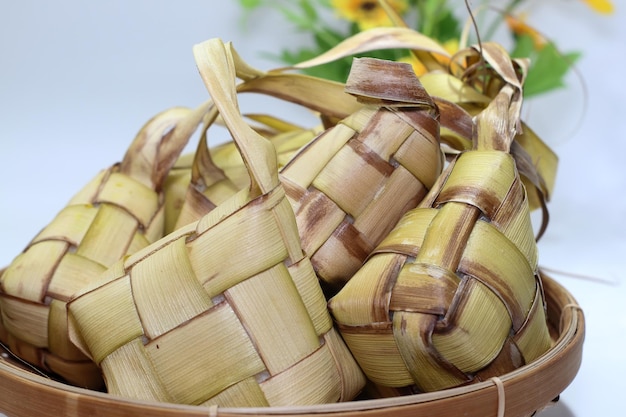The photograph showcases a light beige pot containing a collection of intricate, square-like woven objects. These objects appear to be crafted from tough, strip-like materials, possibly sugar cane or palm leaf, giving them a yellowish-tan color with hints of brown around the edges. The woven items are meticulously interwoven, resembling small containers or baskets. Situated against a light gray background, the pot is complemented by a vibrant plant with lively green leaves and striking yellow flowers with brown centers. The flowers add a touch of color and natural beauty to the composition, creating a harmonious blend of elements in the image.